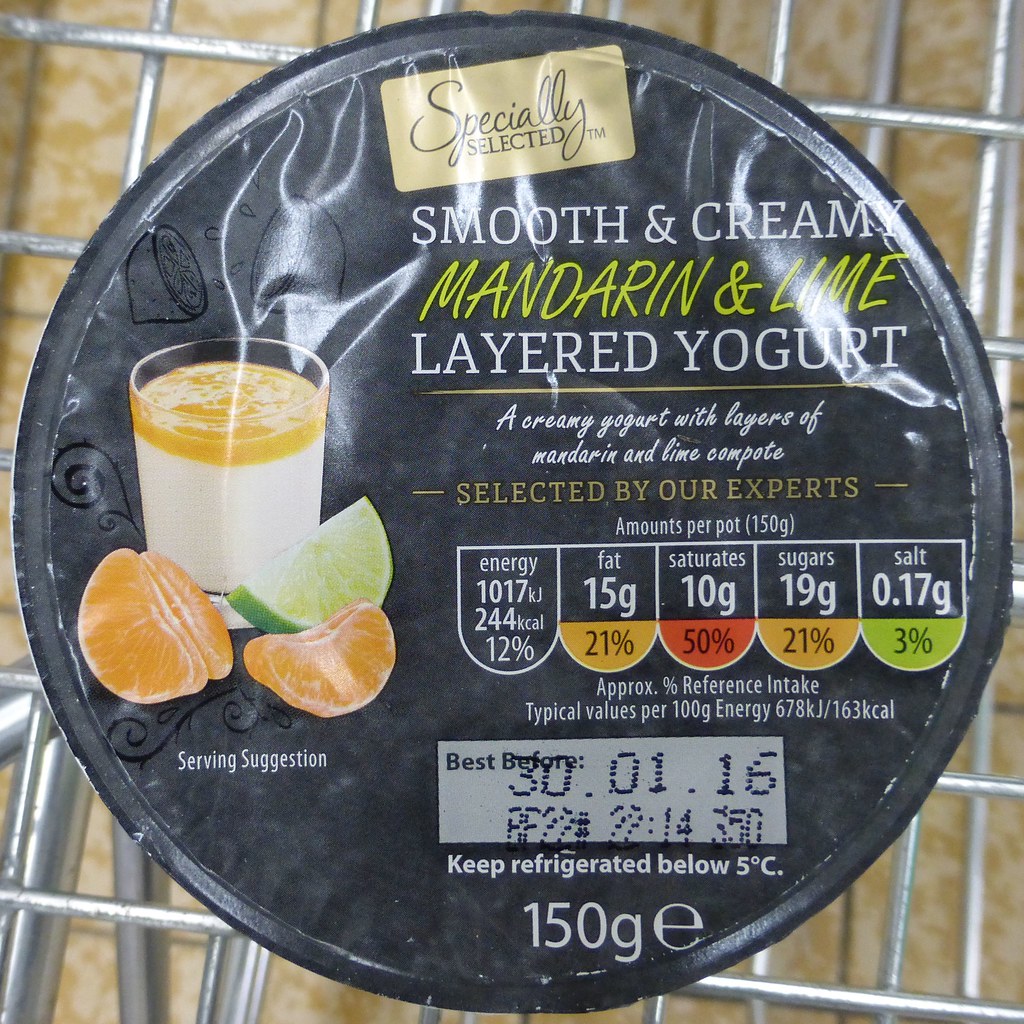The image depicts the top of a yogurt container lid, which is placed on a metal wire mesh reminiscent of a shopping cart. The ground beneath is mottled yellow and white. The lid, which is oval-shaped and black plastic, prominently features the brand name "Specially Selected" in a gold rectangle at the top. The product is described as "Smooth and Creamy Mandarin and Lime Layered Yogurt," and beneath that, it says, "A creamy yogurt with layers of mandarin and lime compote selected by our experts."

The lid includes an illustration showing a glass with a white fluid topped with an orange fluid, adorned with orange slices and a lime wedge. It details nutritional information: each 150g pot contains 1017 kilojoules (244 kilocalories) of energy, 15 grams of fat (21%), 10 grams of saturates (50%), 19 grams of sugars (21%), and 0.17 grams of salt (3%). Additional nutritional information is provided for typical values per 100 grams: 678 kilojoules (163 kilocalories). The best before date is January 30, 2016, and it advises keeping the product refrigerated below 5 degrees Celsius. The background design includes images of peeled mandarin segments and a sliced lime, illustrating the yogurt's flavor profile.